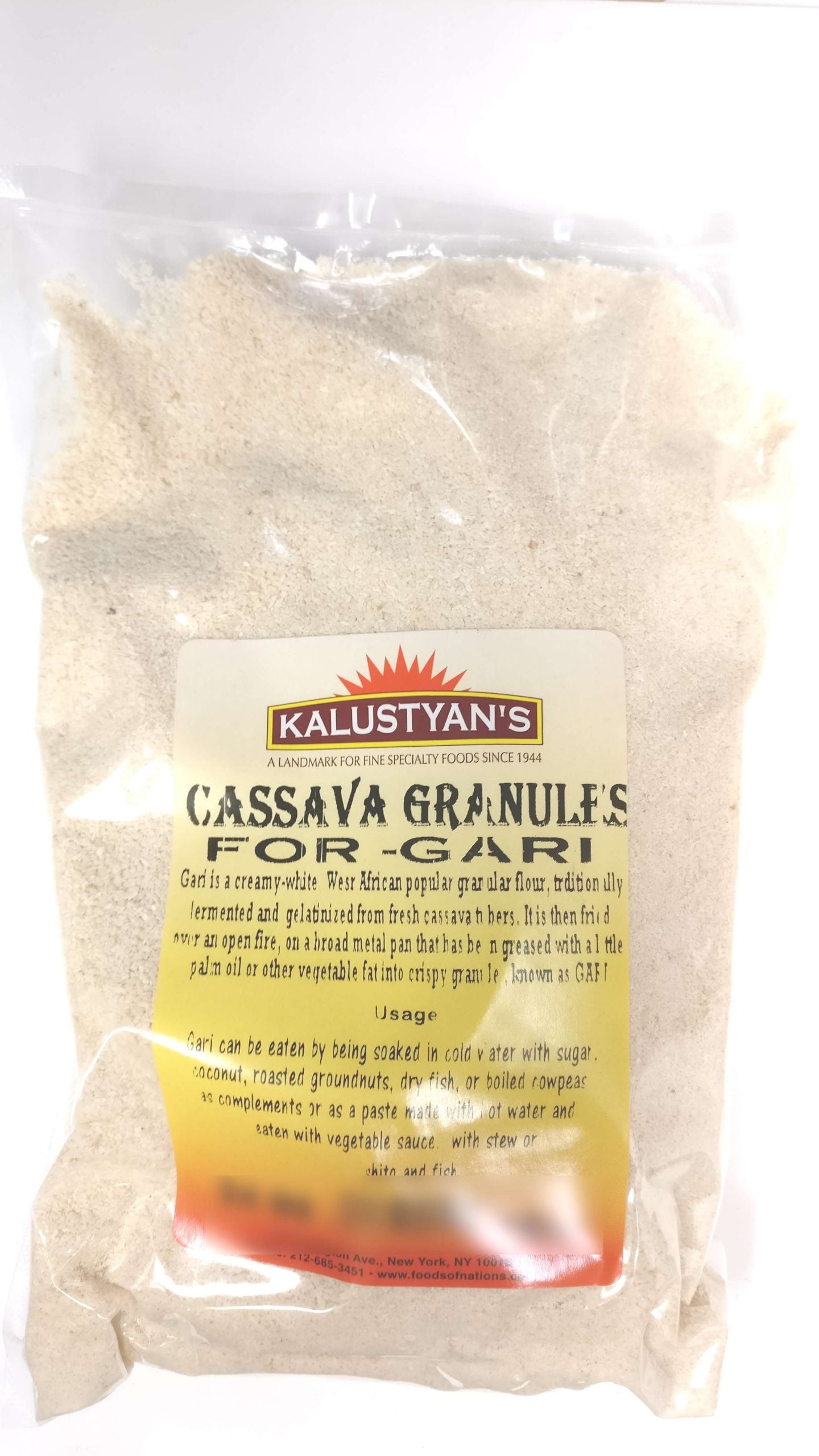This image features a clear, sealed bag filled with tiny white and off-white circular granules, labeled as "cassava granules for Gari." The label starts at the top of the bag and transitions in color from white to yellow to red. Prominently displayed on the front of the label is the brand name "Kalustyan's" in white lettering set within a dark red rectangle. The label boasts the tagline, "A landmark for fine specialty food since 1944." Additional text describes Gari as a "creamy white West African popular granular flour traditionally fermented and gelatinized from fresh cassava." The package includes usage tips, suggesting that Gari can be soaked in cold water with coconut, roasted groundnuts, dry fish, or boiled cow peas, or eaten with vegetable sauce or stew. The bag appears shiny, with some text partially blurred but still conveying the rich cultural and culinary significance of the product.